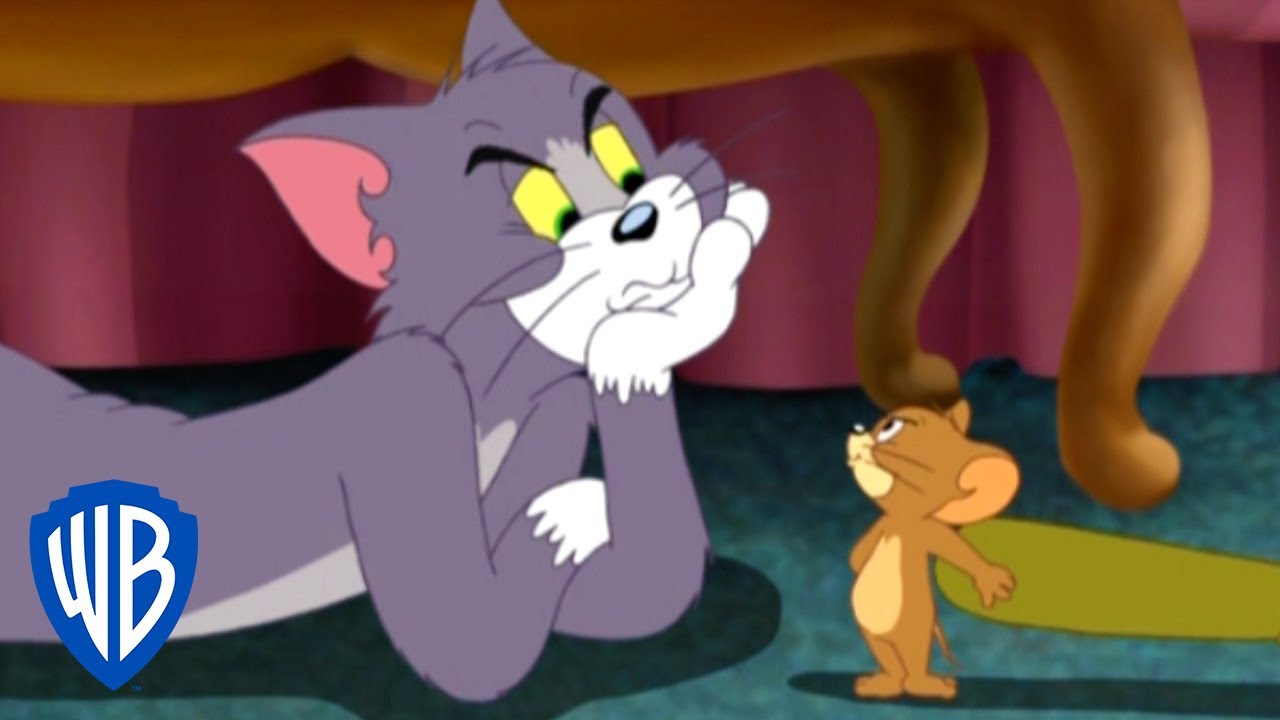This is a detailed still from a Warner Brothers Tom and Jerry cartoon. The iconic Warner Brothers logo with the blue shield and white reverse type resides in the bottom left corner of the image. The scene captures Tom, the gray cat with a white belly, white paws, and a white mask over his snout, under what appears to be a settee with wooden legs. Behind them is a burgundy drape that touches the teal-colored ground. Tom’s yellow eyes, lined with green and black, show a look of annoyance and boredom. His light pink ears are perked, and he rests his head on a hand with his arms crossed in a contemplative manner. To his right, Jerry, the small brown mouse with a lighter-colored belly and snout, stands looking rebellious and angry. Jerry holds an unseen object behind his back, suggesting he's scheming something against Tom as he gestures with one arm. The whole scene unfolds with them nestled under the settee, adding tension and humor typical of the Tom and Jerry series.